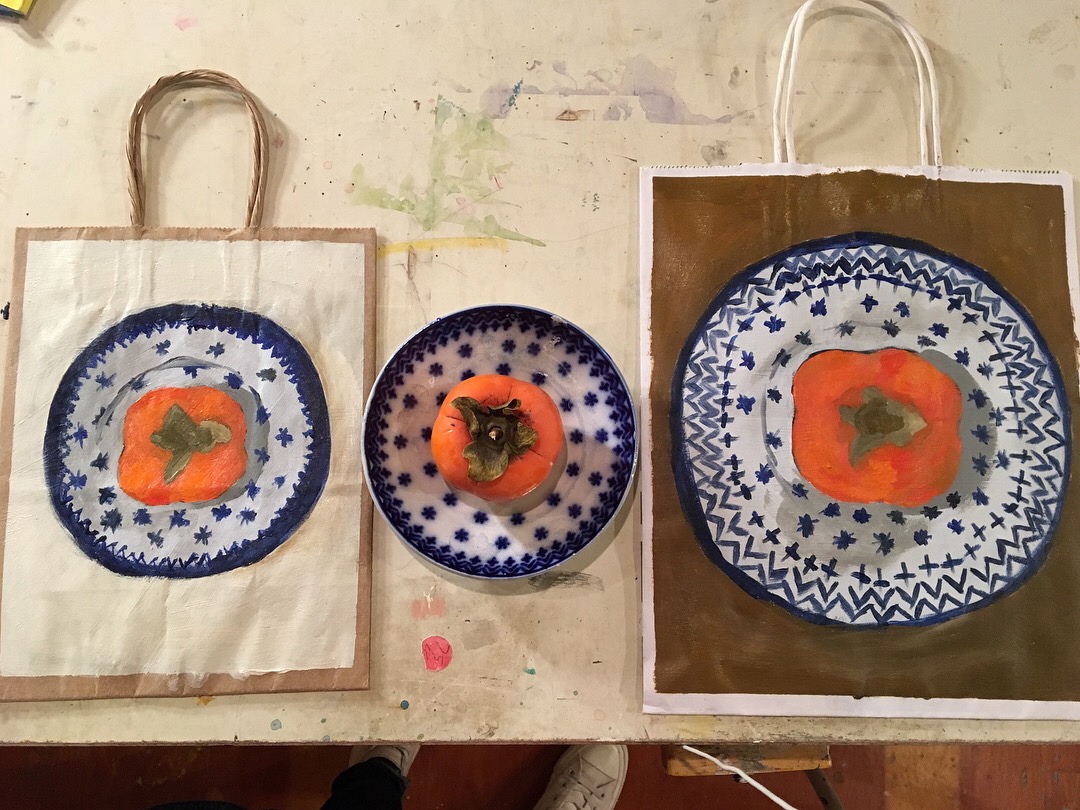This photograph, taken from above, captures a white wooden table splattered with paint stains, suggestive of frequent artistic use. Positioned on the table are two decorated paper bags, one on the left and one on the right. The left bag, light brown with a brown handle, has a piece of white paper taped to its front. The paper showcases a painted design featuring a blue circle with white laurel shapes encircling an orange square and a brown leaf in the center—a possible watercolor or acrylic artwork depicting a plate. Adjacent to this bag, a blue-rimmed shallow bowl sits in the middle of the table. This bowl has a white interior dotted with blue flower patterns and contains a realistic-looking orange tomato with brownish leaves on top. To the right, there is a larger white paper bag with white handles. Its exterior features a brown square with a blue circular pattern of triangles, plus signs, and flower-like dots, similar in style to the left bag's artwork. The center of this design also contains an orange square and a brown leaf, mirroring the aesthetics of the adjacent items. The overall scene portrays a harmonious blend of functional objects and artistic representations, united by the recurring blue and orange theme.